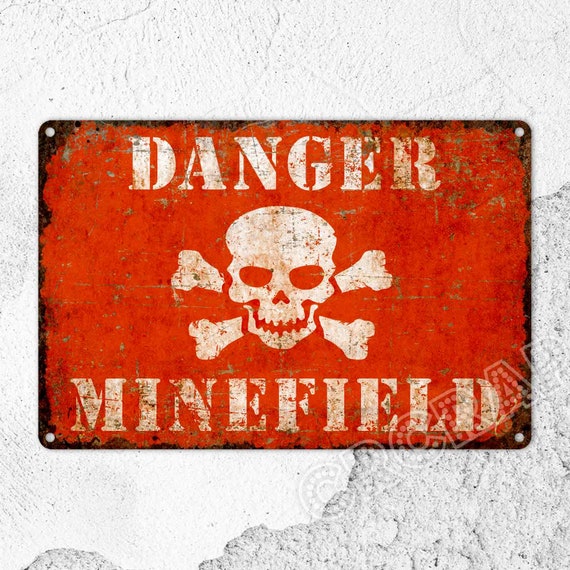The image showcases a close-up of a worn, rectangular plaque mounted on a textured, whitish wall. The plaque, heavily rusted along its edges and marred by scratches, displays bold white text against a distressed red background that reads "Danger Minefield." Central to the warning is a white skull and crossbones symbol, positioned prominently between the text. Each of the plaque's four corners features a hole, further emphasizing its aged and weathered condition. The surrounding wall, possibly made of plaster or stone, adds to the historical feel of the scene with its cracks and uneven texture. No additional objects or people are visible in the image, focusing attention solely on the ominous and battle-worn warning sign.